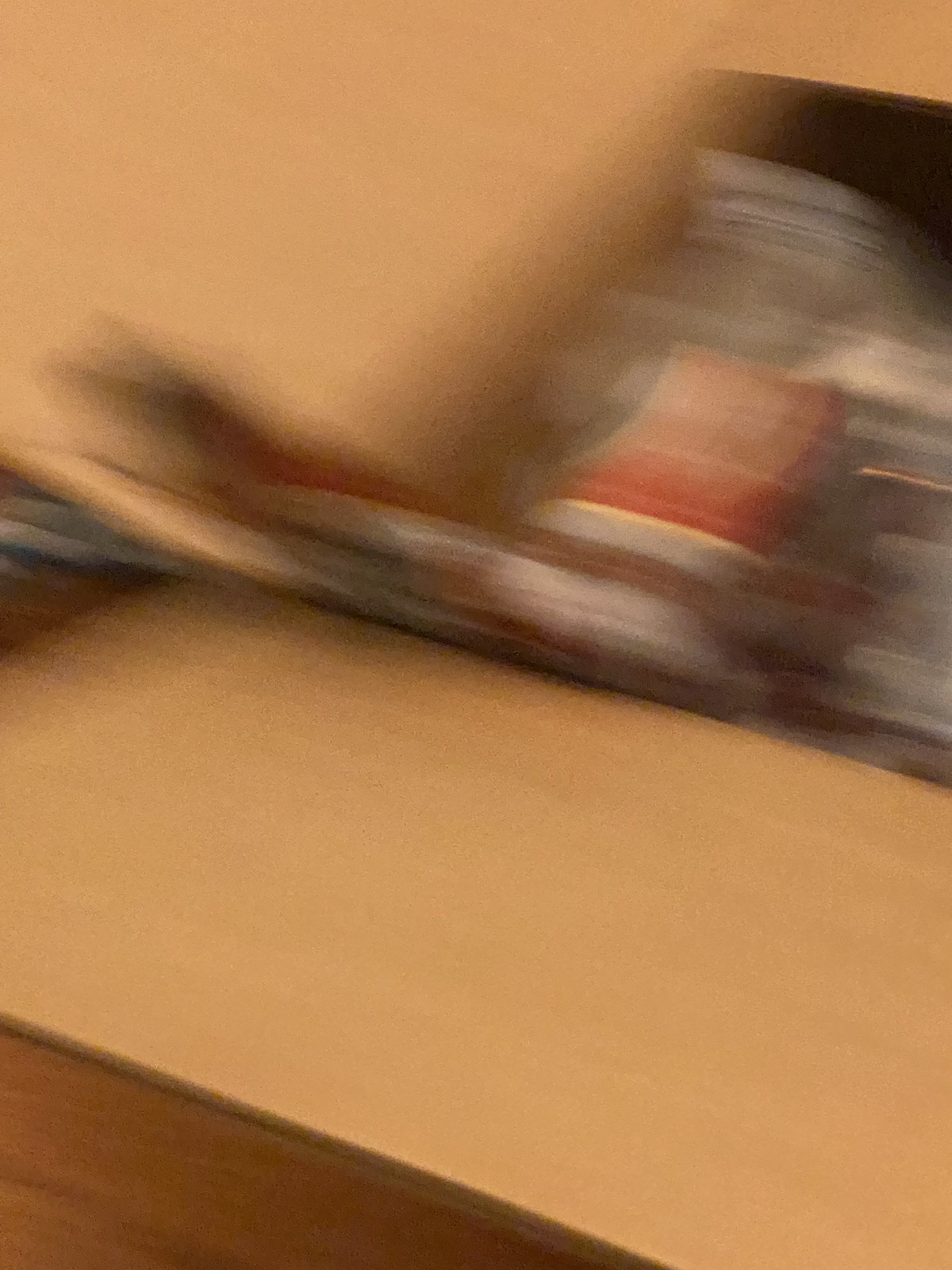This is a highly blurred color photograph, making it difficult to discern specific objects. Dominating the image are tan, brown, red, and white hues. A large tan shape, appearing U-shaped, is prominent in the upper left corner, extending across the top and partially down the right side; it might be a hand or part of a cardboard box flap. Below, in the foreground, a dark brown patch suggests a wooden table partially covered by this tan element. Amid these shapes, scattered silver, red, gold, and white colors hint at various items possibly inside the box. The overall scene remains indistinct due to the blur.